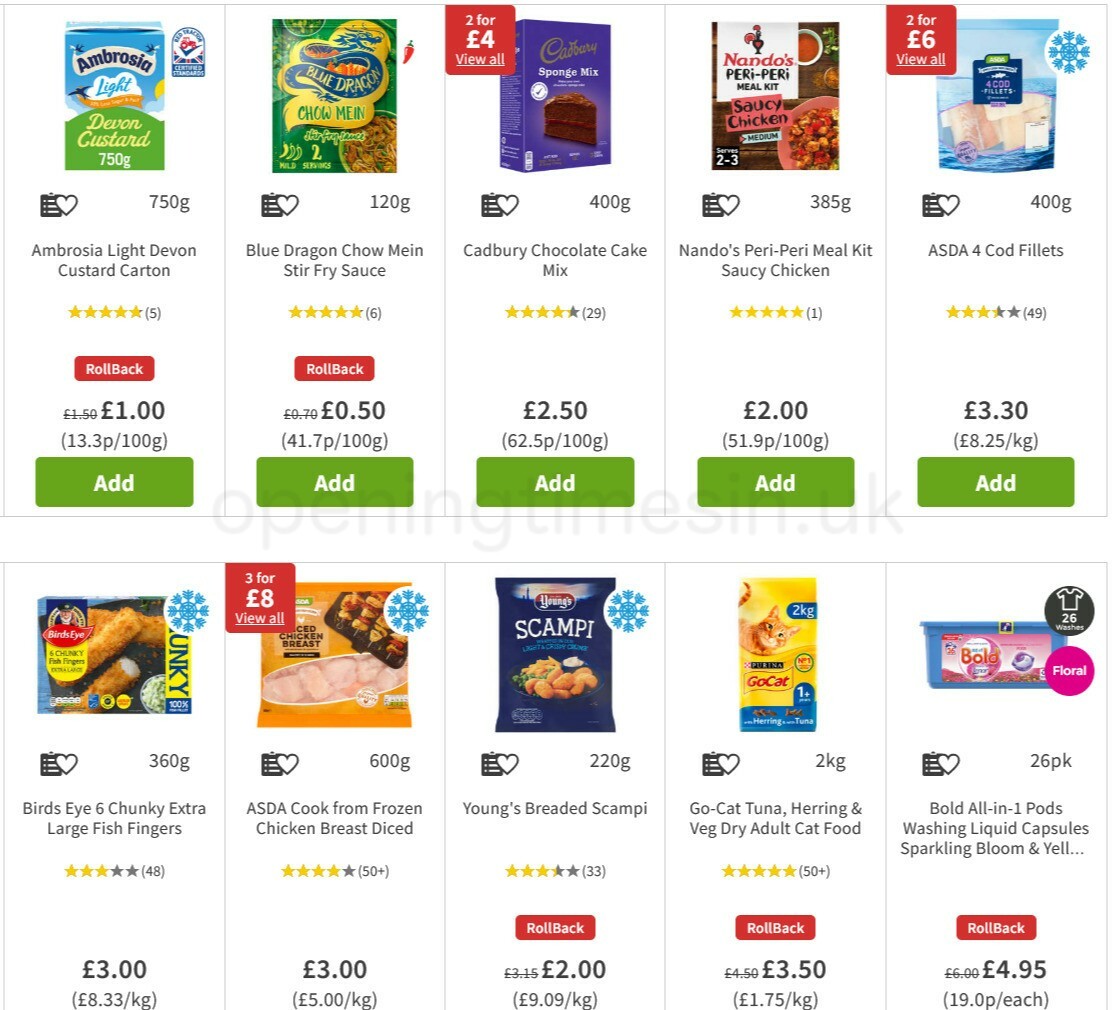This image depicts a webpage that resembles the layout of a supermarket's online shopping interface, likely associated with Walmart, given the presence of "rollback" labels on some items—a signature Walmart promotional feature. The webpage appears to be tailored for an overseas market, showcasing prices in British Pounds (£) instead of US Dollars ($). The display features ten diverse grocery items available for online purchase. 

Prominently listed items include:
1. Ambrosia Devon Custard priced at £1.00, with options to add to the cart or mark as a favorite.
2. Blue Dragon Chow Mein Stir-Fry Sauce at £0.50.
3. Cadbury Chocolate Cake Mix for £2.50.
4. Nando's Peri-Peri Meal Kit priced at £2.00.
5. Cod Fillets available for £3.30.
6. Bird's Eye Chunky Extra-Large Fish Fingers for £3.00.
7. Cooked-from-frozen Diced Chicken Breast at £3.00.
8. Young's Breaded Scampi priced at £2.00.
9. Go-Cat Tuna, Herring, and Veg Dry Adult Cat Food for £3.50.
10. Bold All-in-One Laundry Pods at £4.95.

Each item includes a clickable button for easy addition to the shopping cart, enhancing user convenience. The webpage's intuitive design aims to streamline the shopping experience, confirming it as a potential checklist for household essentials.